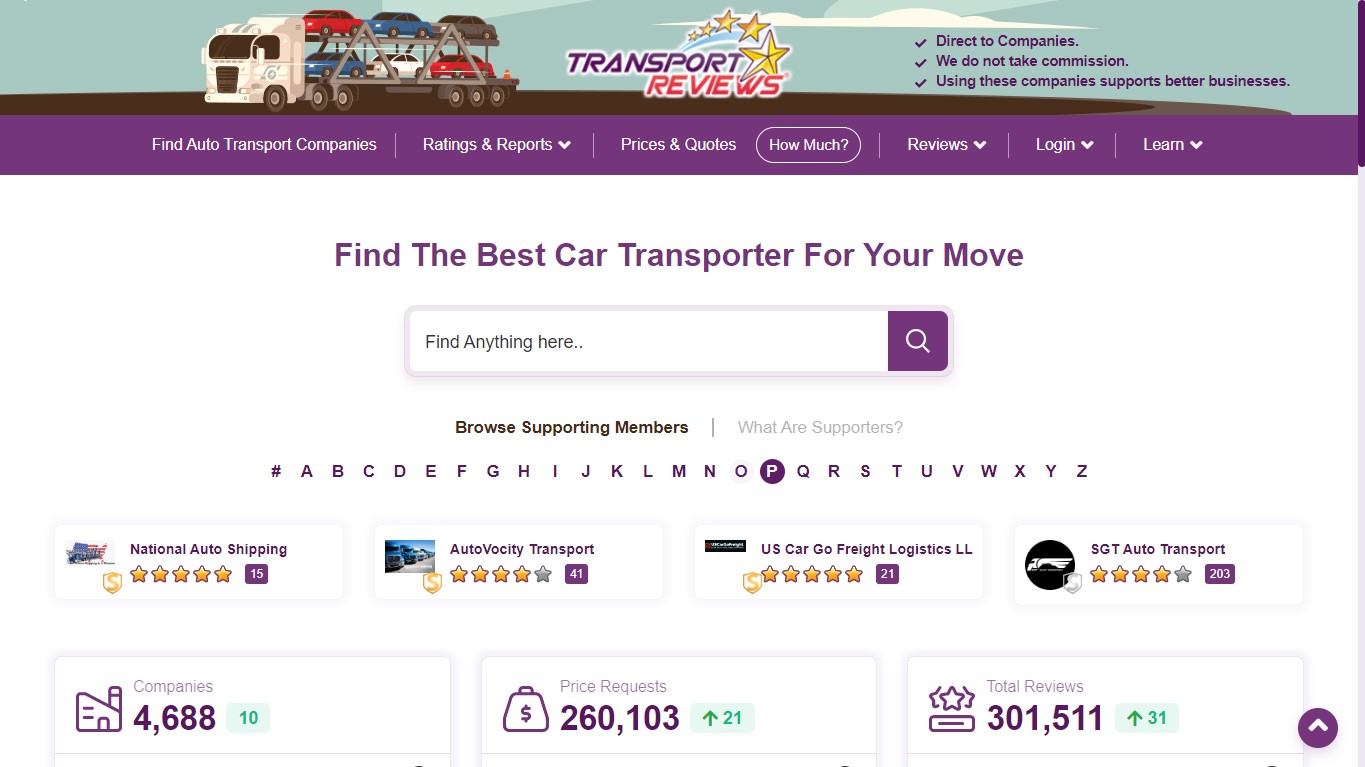A screenshot of the Transport Reviews website provides an in-depth look into its features and interface. Dominating the visual is a large image of an 18-wheeler car carrier, holding six stacked cars. Highlighted prominently is a statement asserting, "Direct to Companies, we do not take commissions," encouraging users to support better businesses through their choices.

The top navigation menu, styled in purple, includes options for discovering transport companies, ratings and reports, prices and quotes, and contains a white-outline button labeled, "How much?" Against the purple background, buttons for Reviews, Logins, and Learn are also visible. A call-to-action invites users to "Find the best car transporter for your move," which accompanies a search field with a purple search button.

Under the prompt "Browse Supporting Members," the displayed alphabet features the letter 'P' highlighted. Below this, four transport companies are listed: National Auto Shipping, Vosity Transport, U.S. Cargo, Freighter, Logistics, LLC, and SGT Auto Transport. Their respective ratings are shown: two companies have five-star ratings, while the remaining two have four-star ratings.

Further down, statistical details are presented alongside icons—a factory icon indicating "Companies: 4,688," a money bag icon representing "Total Requests: 260,103," and a star icon showing "Total Reviews: 301,511."